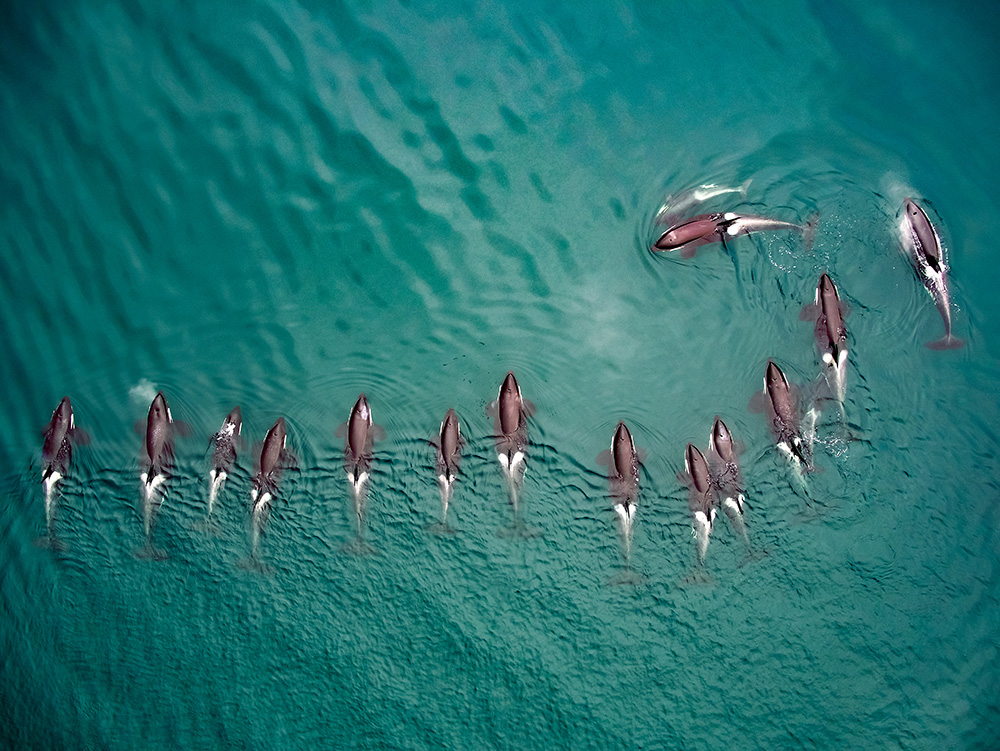This stunning aerial photograph showcases a serene, turquoise ocean with a school of fifteen orcas gracefully swimming in a line. The calm, rippling waters appear almost greenish-blue, providing a stark contrast to the orcas' striking black and white coloration. Captured from a bird's-eye view, presumably from a helicopter, the orcas move left to right, with several beginning to curve upward, hinting at a change in direction. Among the orcas, some appear to be younger, adding a familial touch to the scene. Overall, the image beautifully captures this harmonious, natural spectacle in striking detail.